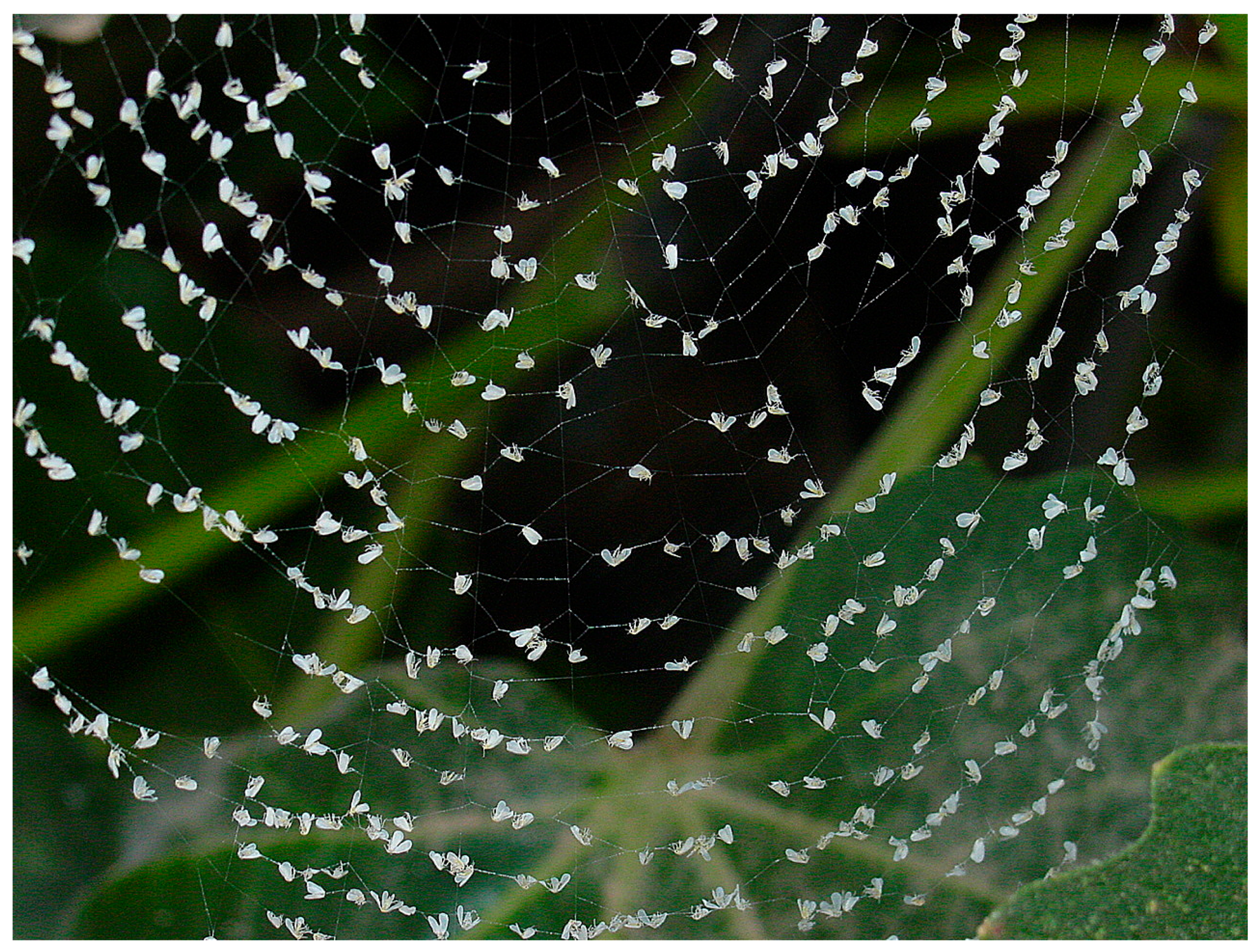This nighttime photograph captures a large spiderweb densely populated by a couple hundred tiny white insects, likely midges or small flies, framed against a backdrop of dark pitch-black sky. The web, intricately spun in front of a green plant with broad leaves and visible stems, glistens with the encased bodies of the insects. Some of these insects appear to be wrapped in silk, evidence of the spider's industrious feeding habits, while others remain untouched but entangled in the web. The green plant, partially visible across the photo, adds a contrasting natural element to the scene. Despite the overwhelming number of tiny captured insects, every strand of the spiderweb remains discernible, showcasing its delicate yet effective construction in nature's ongoing drama.